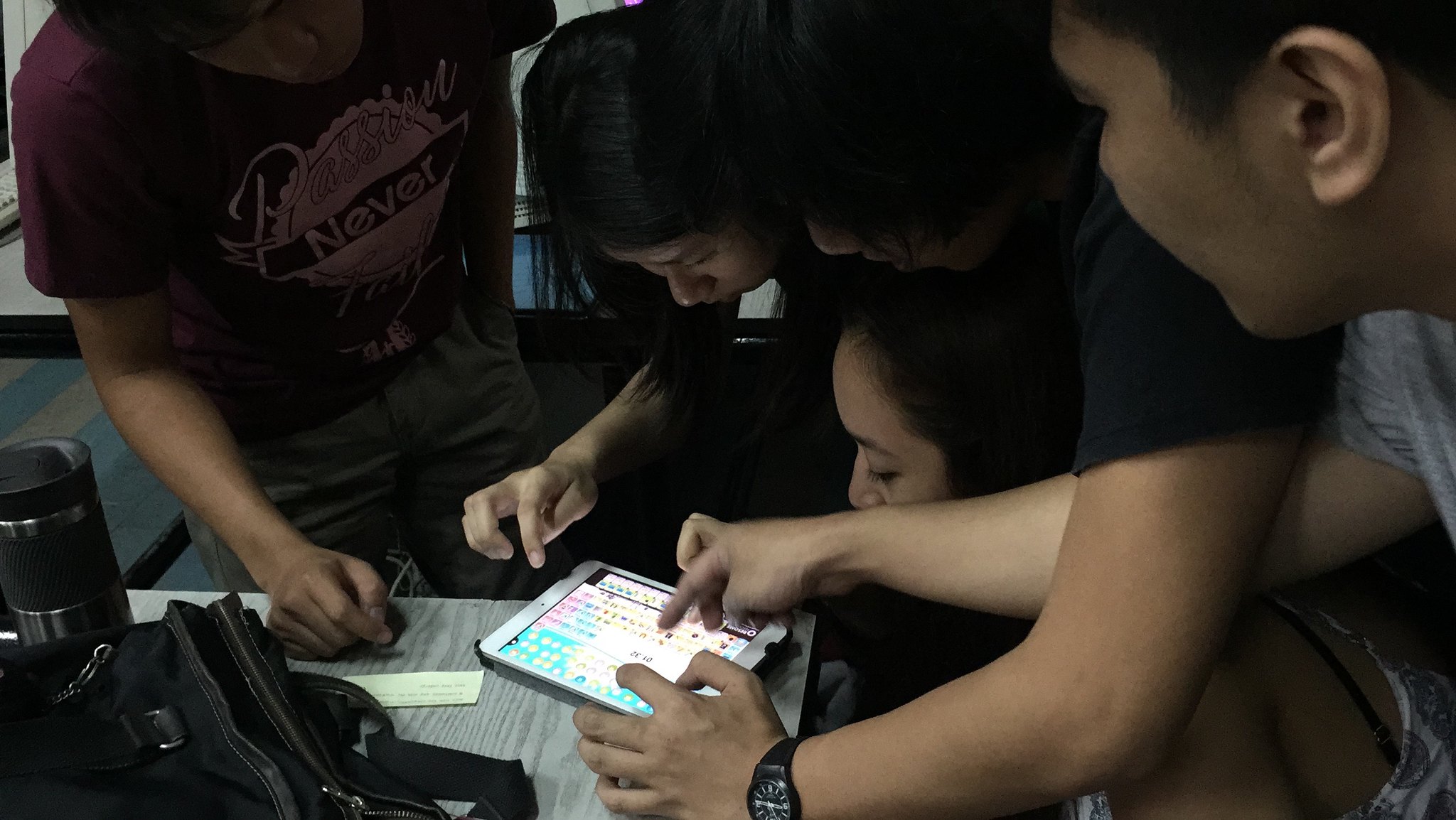In a dimly lit photograph, a group of five young, predominantly Asian individuals are gathered around a small, light wood-colored table, intently focused on a tablet screen that is busy with information. Three of the individuals are actively swiping or touching the screen, while another stands ready to interact. The scene is dark, making it difficult to discern every detail, but one person wearing a marine-colored shirt with the words "Never" and "Passion" in different fonts stands out. Another individual is identifiable by a black short-sleeved t-shirt and a black wristwatch on his left hand, which is resting on the table as he reaches towards the tablet. The group appears to be engaged with what seems to be a game or application displaying complex visuals. Aside from the tablet, the table holds a thermos and possibly some bags, adding to the clustered and somewhat chaotic ambiance of the scene.